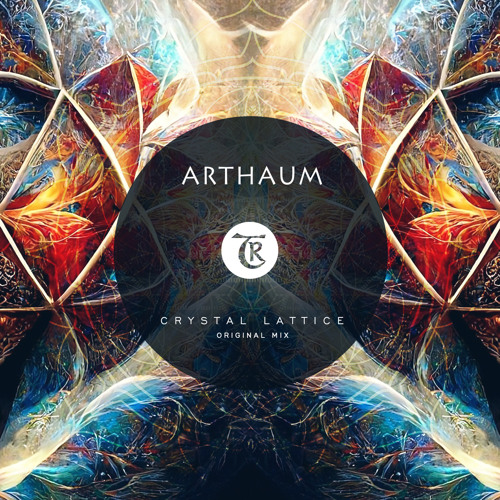The image is a modern, full-color design likely for a vinyl disc cover or an advertisement, displaying the text "ARTHAEUM" in all capital letters at the top. Below, it reads "Crystal Lattice Original Mix" inside a large central black circle resembling a record, enhanced by a smaller white circle in its center and a stylized calligraphy "T" intertwined with a capital "R." The cover features an abstract, visually striking background with vertical symmetry, where the left and right sides mirror each other. It includes a vibrant array of paint swashes, fractal patterns, and a mysterious network of geometric shapes outlined in off-white hues. The intricate background combines an array of colors such as bright blue, green, fuchsia, red, yellow, orange, and gray, creating a dynamic and artsy yet cohesive image that draws attention to its modern and eclectic design.